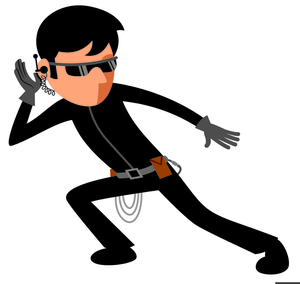This image is a computer-generated character drawing of a spy, reminiscent of a James Bond figure. The background is plain white, keeping the focus solely on the central figure. The man, dressed in a sleek black bodysuit, leans slightly to his right, bending his right knee and extending his left leg behind him, balanced on his tippy toe. His right arm is bent at the elbow, with his hand up to his ear, suggesting he is receiving communication through a visible black earpiece. He has short black hair and wears black sunglasses with gray trim. 

The spy's outfit includes gray gloves and a single-piece suit adorned with a thin gray stripe down the front. A gray belt wraps around his waist, featuring additional spy gear, such as two brown patches on either hip and three silver chains or ropes hanging on one side. The figure's right hand is near his ear, while his left arm extends straight out to the side. Despite the simplicity of the drawing, the figure is identifiable by his distinct black hair, glasses, and the notable absence of a mouth, save for a visible nose. This detailed attire and posture effectively convey the essence of a stealthy, high-tech operative.